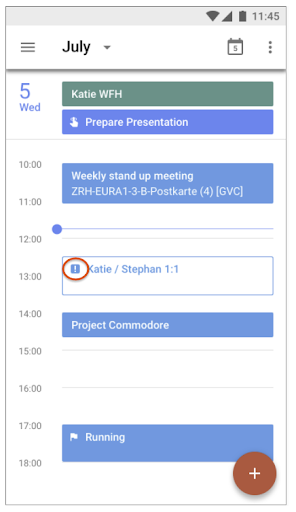The screenshot captures a daily agenda for Wednesday, July 5th. At the top of the image, the month "July" is displayed alongside a calendar icon, followed by the date "5 Wed," indicating Wednesday. Below this, there's a green rectangular section labeled "KCWFH," along with a blue rectangular section titled "Prepare Presentation."

The schedule starts with a "Weekly Stand-Up Meeting" from 10:00 to 11:00 AM, with a unique meeting code "ZRH-EUR-13BPROSKATES." A horizontal line extends from 11:00 AM and has a circle on the left side, continuing downwards. From 12:00 PM to 1:00 PM, an outlined blue rectangle features a notation, "KT-Stephanie 1:1."

In the afternoon, from 2:00 PM to 3:00 PM, the schedule includes "Project Komodo." The slots from 3:00 PM to 4:00 PM and 4:00 PM to 5:00 PM are blank. From 5:00 PM to 6:00 PM, the agenda lists "Running." At the bottom of the page, there's a plus sign icon for adding new events or tasks.